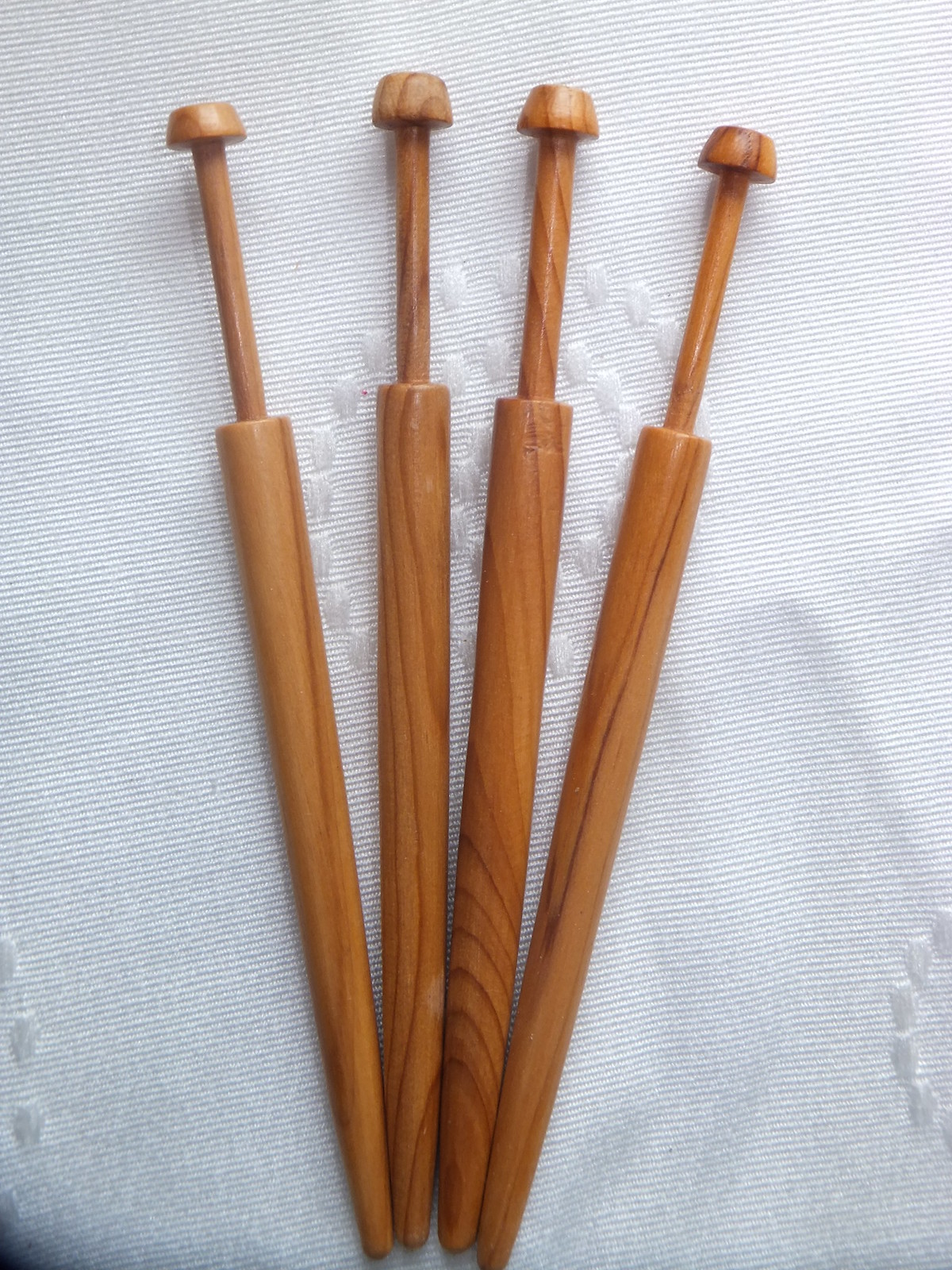The photograph shows four finely sanded, handcrafted wooden objects arranged side by side in a fan pattern on a white tablecloth with an embroidered spiral pattern. Each object is made of light to medium brown wood with a visible grain, and they appear to be a form of dowel or pin, featuring a distinctive handle on one end that is slightly wider and a main shaft that extends outward, ending in a dull point. The wood is meticulously finished, suggesting that these might be self-made hobby projects, possibly intended for use as training blades or decorative rolling pins. The uniform craftsmanship and elegant presentation on the fabric evoke an impression of a product display, potentially for resale.